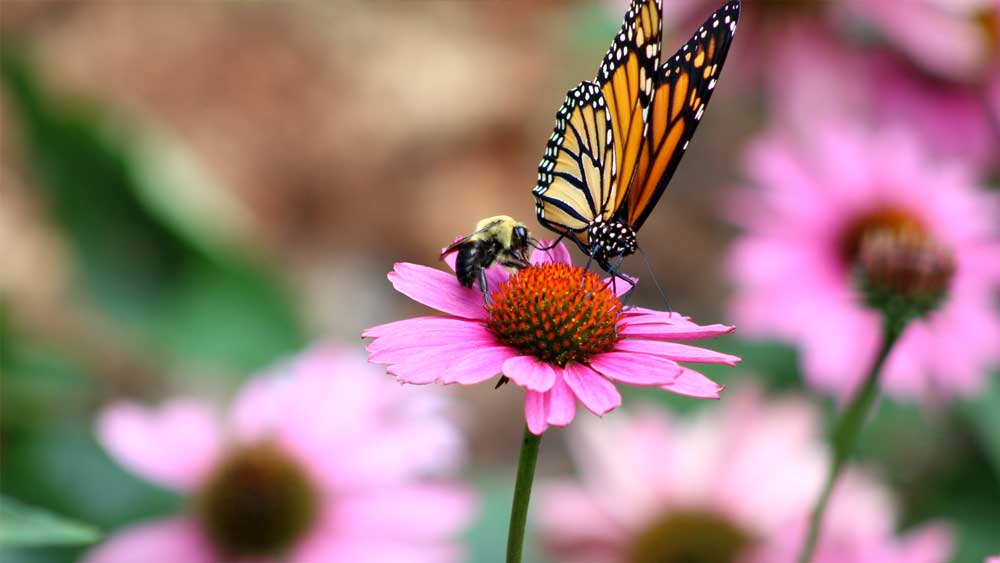In this detailed outdoor photograph, the central focus is a vibrant pink flower with a prominent orange center and green accents. Perched atop this flower is a striking monarch butterfly, characterized by its orange wings adorned with black lines and white spots. Adjacent to the butterfly, a charming bumblebee with a black and yellow body is also visible. Both insects appear to be collecting pollen from the colorful flower. The background features a high depth of field, resulting in a beautifully blurred backdrop filled with similar pink and orange flowers, enhancing the main subjects' prominence. The setting appears to be a field or garden, creating a natural and serene atmosphere with a palette including shades of pink, orange, green, and touches of black and white.